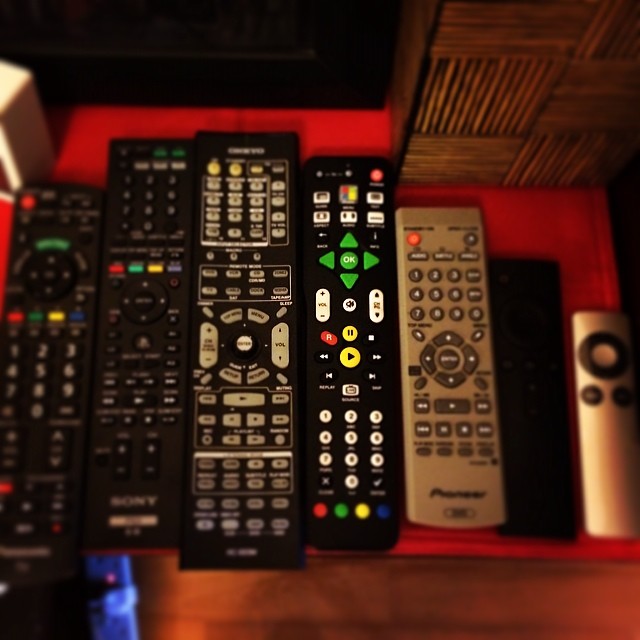In this detailed photograph, there is an assortment of seven remote controls of varying sizes meticulously laid out on a red cloth that drapes over a wooden surface, which appears to resemble a normal distribution curve. The four remotes on the left are black, each studded with a colorful variety of buttons in red, green, blue, yellow, and white. The fifth remote, positioned to the right of these black remotes, is distinctly grey and branded by Pioneer, featuring dark grey buttons. Adjacent to this grey remote is a sleek, black remote, likely for an Amazon Fire Stick, which seems to blend into the background. The furthest right remote is a sophisticated silver Apple device with an iconic, black circular control. In the background, a wooden TV stand is visible, supporting the lower part of a black television within its frame. To the far right of the TV, there's a rectangular ornament made of small, wooden crisscrossing tiles, adding a rustic aesthetic to the setting. The red cloth over the reddish-brown laminate flooring contributes a vibrant touch to the overall warm, homey atmosphere depicted in the image.